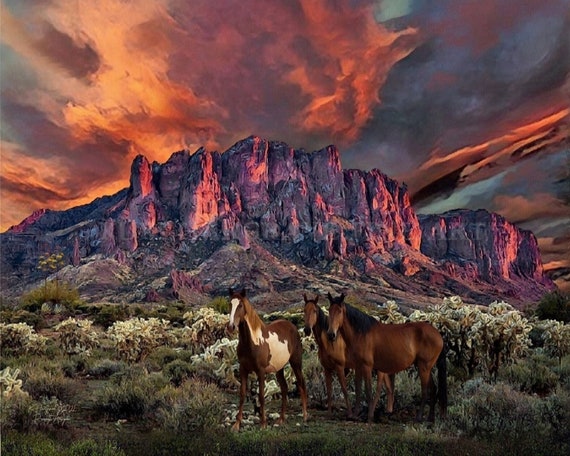This surreal painting, possibly set during a fiery southwest sunset, depicts a dramatic rocky mesa, likely a butte, prominently rising in the background. The sky is an explosion of colors, with reds, purples, peaches, and yellows blending into a dark blue-green expanse, resembling a wild oil painting with splotchy clouds. In the foreground, amidst lush green and yellowish-green grasses and shrubberies, stand three wild horses. Two are chestnut brown with black manes and tails, while the third is similarly colored but adorned with distinctive white patches on its belly, neck, and forehead. The horses are all gazing towards the viewer, adding to the captivating, almost lifelike feel of this mesmerizing southwestern U.S. desert landscape. The light from the sunset casts a mesmerizing blend of pink, purple, and red hues on the mesa, enhancing the painting's otherworldly aura.